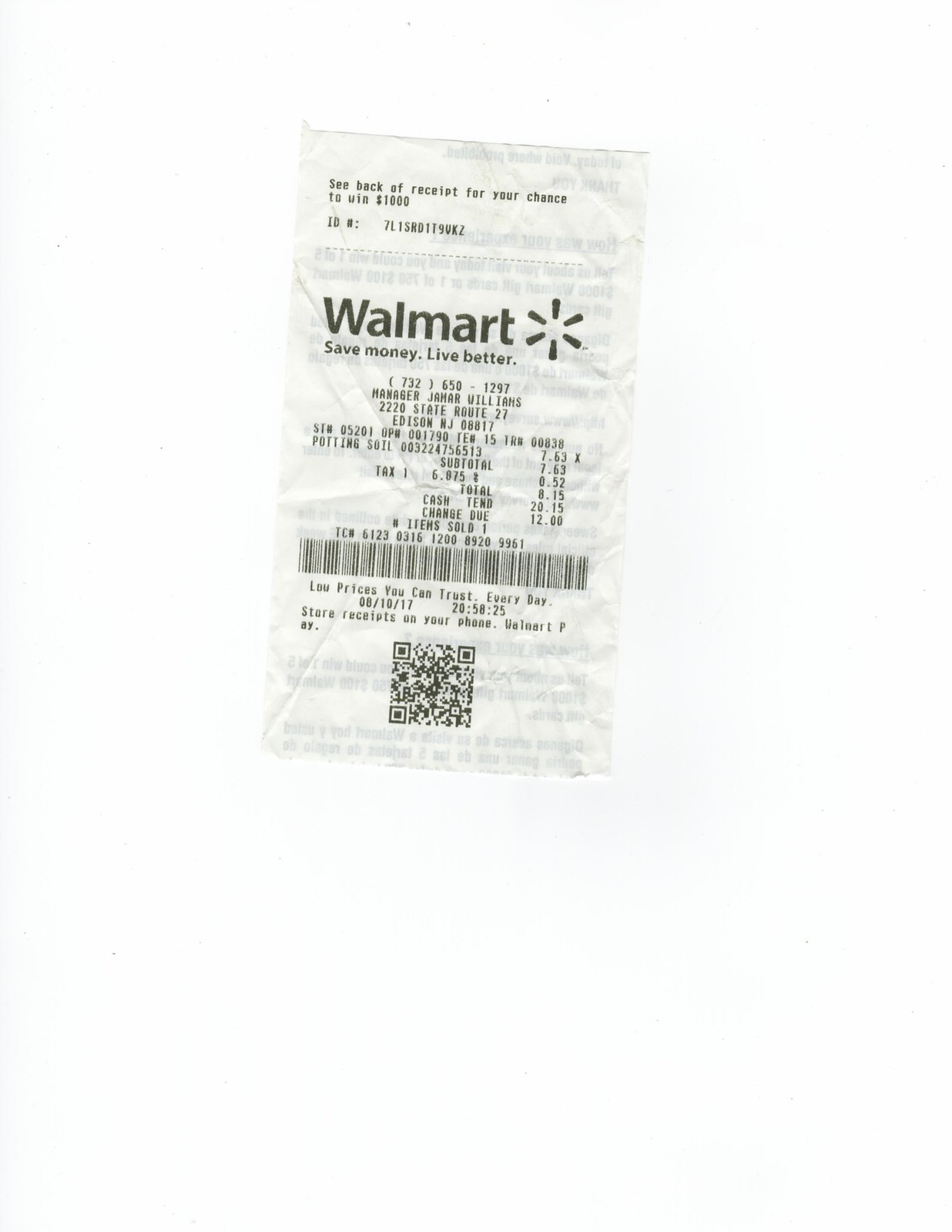The image depicts a slightly crumpled and worn Walmart receipt, likely retrieved from an enclosed space like a pocket. The receipt's white paper shows signs of age and wear. At the very top, in prominent black lettering, it reads "See back of receipt for your chance to win $1,000." Below this, an ID number "7L1SRD119UK2" is printed. The receipt boldly displays "Walmart" along with their slogan, "Save money, live better," followed by the phone number "(732) 650-1297." The manager’s name, Jamar Villains, appears underneath, along with the store address: "200 State Route 27, Edison, NJ 08817." 

The purchase details reveal that the customer bought a pot and soil for $7.63. They paid with a $20 bill and received $12 in change. Additionally, the receipt includes a QR code at the bottom.